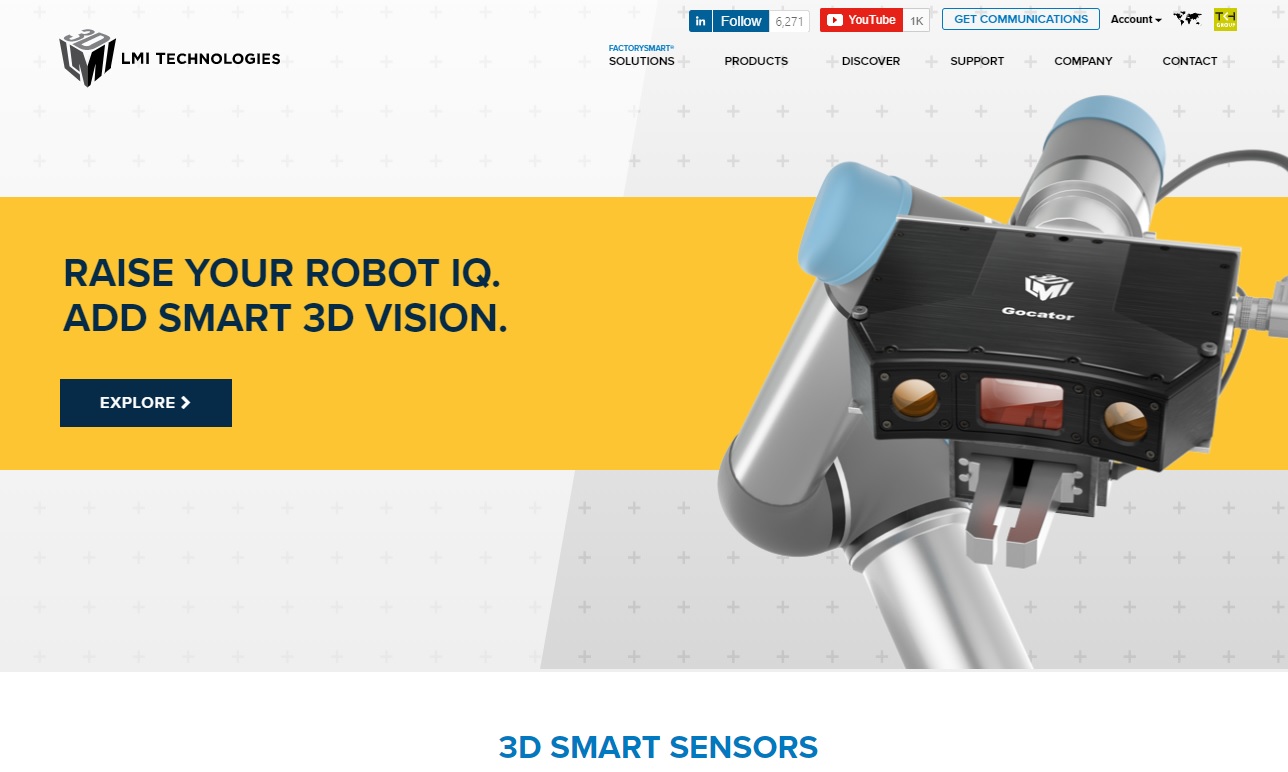The webpage for LMI Technologies offers various ways to contact the company, including links to their YouTube channel. In the middle of the page, a horizontal mustard-colored panel features a call to action in dark text, stating, "Raise Your Robot IQ: Add Smart 3D Vision," accompanied by an "Explore" button. The image on the page showcases what appears to be a robotic arm, colored in silver and blue, with a black device clamped onto the front of it. The device features screens and is labeled "Geocator," suggesting it is likely a sophisticated piece of technology aimed at enhancing robotic functionality.